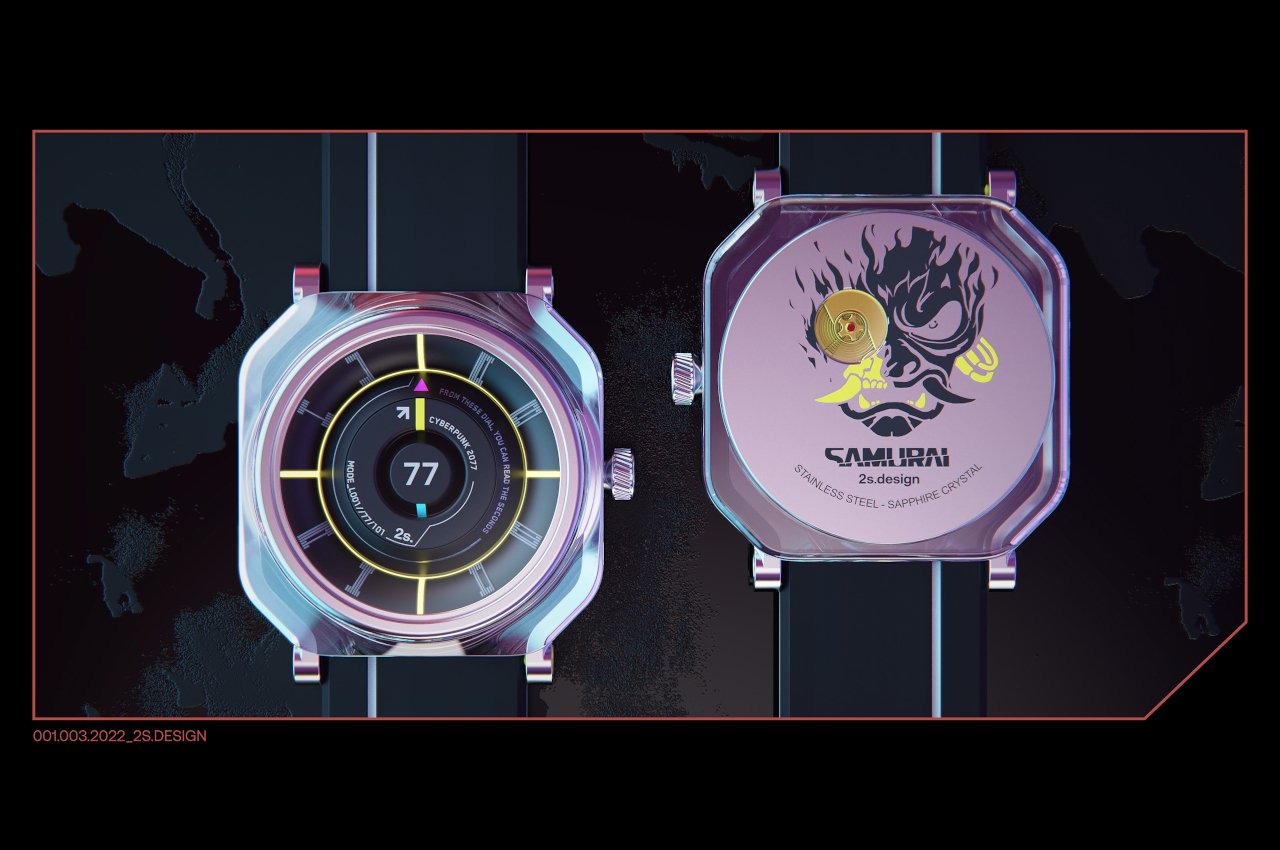This mock-up advertisement features a detailed image showcasing both the front and back of a conceptual Cyberpunk 2077-themed watch. The left side of the image presents the watch's face, highlighted by a prominent number "77" centered within a black circle. The watch face is characterized by a striking metallic purple color with digitized futuristic numerals encircling it. A small yellow line and an orange triangle add further intricate details around the edge. The black strap of the watch is accented by a light blue stripe running down the left side.

On the right side of the image, the back of the watch is revealed in a bright, shiny purple hue. It features an elaborate, fiery demonic face design, often interpreted as a samurai with tusked horns, one eye replaced by a silver star. Surrounding the illustration are the words "Samurai 2S Design, Stainless Steel, Sapphire Crystal," underscoring the watch's premium materials and craftsmanship. This dual presentation emphasizes both the bold aesthetic and high-quality materials envisioned for this edgy, Cyberpunk-inspired timepiece.